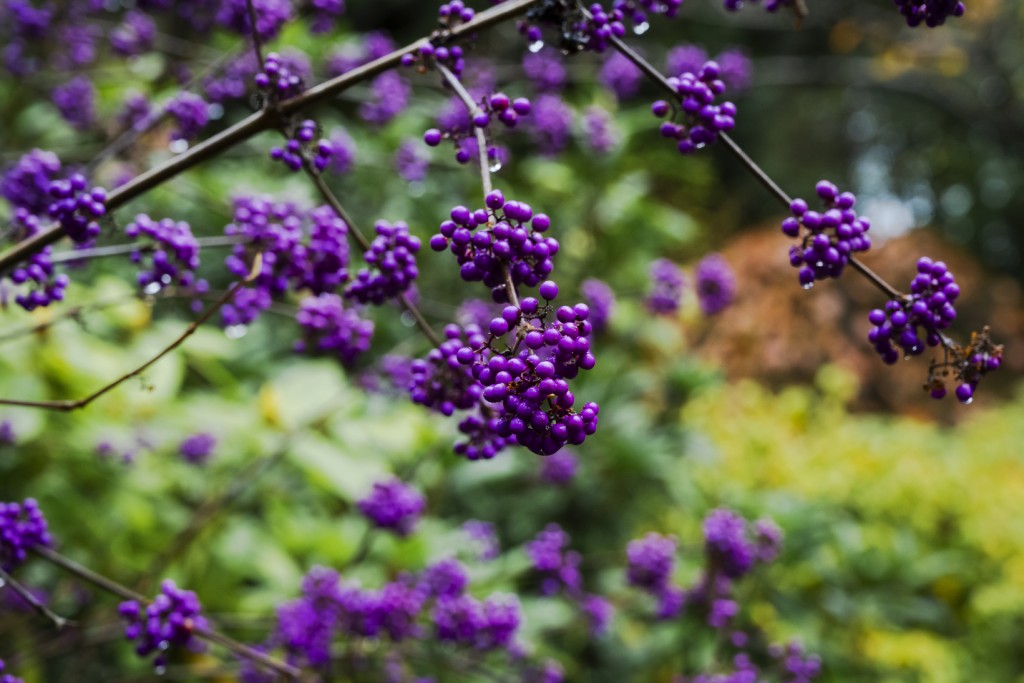This vibrant color photograph captures a close-up view of clusters of bright purple berries, likely beauty berries, hanging from thin branches and twigs. The central focus is on a small series of branches, with each branch supporting densely packed, round berries that glisten with water droplets, suggesting a recent rain. The image's background features a blurred, narrow depth of field filled with dozens of similar purple globs, indicating an abundance of these berries in the half-garden, half-forest setting. The greenery in the backdrop along with hints of orange and possibly decayed brown foliage adds to the natural ambiance. The photograph emphasizes the vividness and uniqueness of the purple berries amidst a hazy, rain-kissed environment.